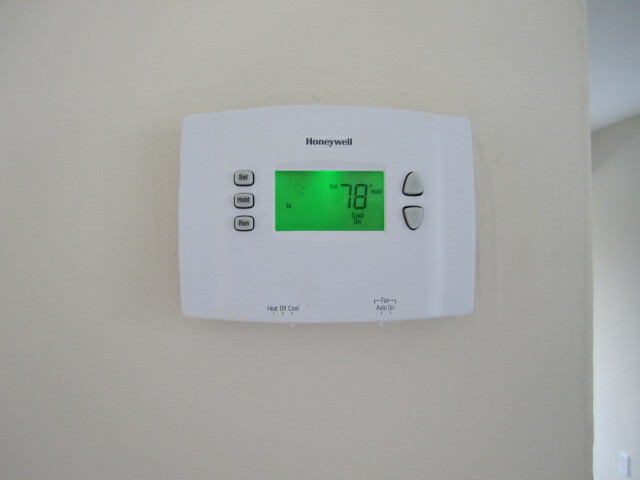This photograph captures a compact Honeywell thermostat, commonly found in homes and apartments. The thermostat features a sleek rectangular design with the Honeywell brand name displayed at the top in small dark navy blue text. 

On the bottom left of the device, there are three distinct settings: "Heat," "Off," and "Cool," allowing users to switch between heating, turning the system off, or cooling. On the bottom right, there is a fan setting with two options labeled under brackets: "Auto" on the left and "On" on the right. The "Auto" setting automatically activates the fan based on the preset temperature, while the "On" setting keeps the fan running continuously regardless of the temperature.

In the middle right area of the thermostat, there are up and down arrow buttons used to adjust the temperature settings. 

Additionally, the top left button is labeled "Set," the central button is labeled "Mode," and the bottom left button is labeled "Run."

The device features a bright green screen displaying the current temperature of 78 degrees Fahrenheit. This screen can show either the ambient room temperature or the set temperature, providing a clear and convenient readout.